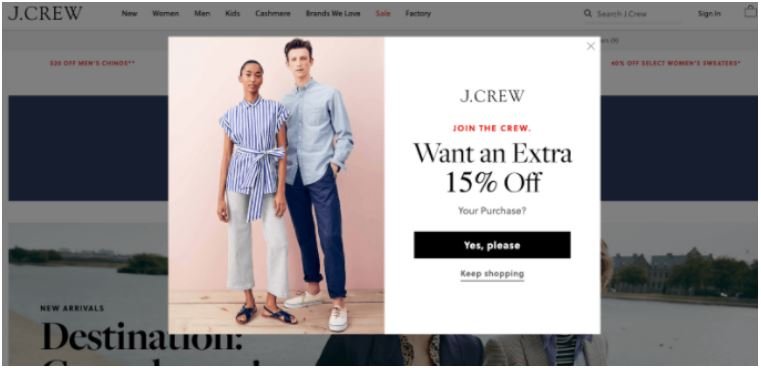This is an annotated screenshot depicting an offer pop-up on the J.Crew website. The main website's interface is visible but darkened to emphasize the pop-up. 

- **Header Section**: A white header spans the top of the page. On the left, "J.Crew" is written in bold black. To the right, navigational sections—"New", "Women", "Men", "Kids", "Cashmere", "Brands We Love", "Sale" (highlighted in red), and "Factory"—are listed in bold black text. Adjacent to these, the search bar labeled "Search J.Crew" with a magnifying glass icon is placed. Continuing to the right, "Sign In" is noted in black text, with a shopping basket icon to its right.
- **Main Webpage**: The obscured background image shows a serene lake with a distant shoreline dotted with houses. Above this image, a dark blue bar is present.

- **Pop-up Details**:
  - **Left Side**: Features a photograph of two individuals standing on a light wooden floor against a pink wall—a woman on the left and a man on the right.
  - **Right Side**: With a white background, the J.Crew logo appears centered at the top in gray text. Below, "Join the Crew" is in bold red, capitalized letters. The primary offer text, "Want an extra 15% off?", is prominently displayed in large black text. Accompanying this offer in smaller text is "Your Purchase".
    - **Call to Action**: A black button with white text "Yes, Please" invites user engagement.
    - **Additional Option**: Underlined black text encourages users to "Keep Shopping".

This accurately captures the visual hierarchy and layout of the website's pop-up offer, ensuring all elements are well-detailed and described.